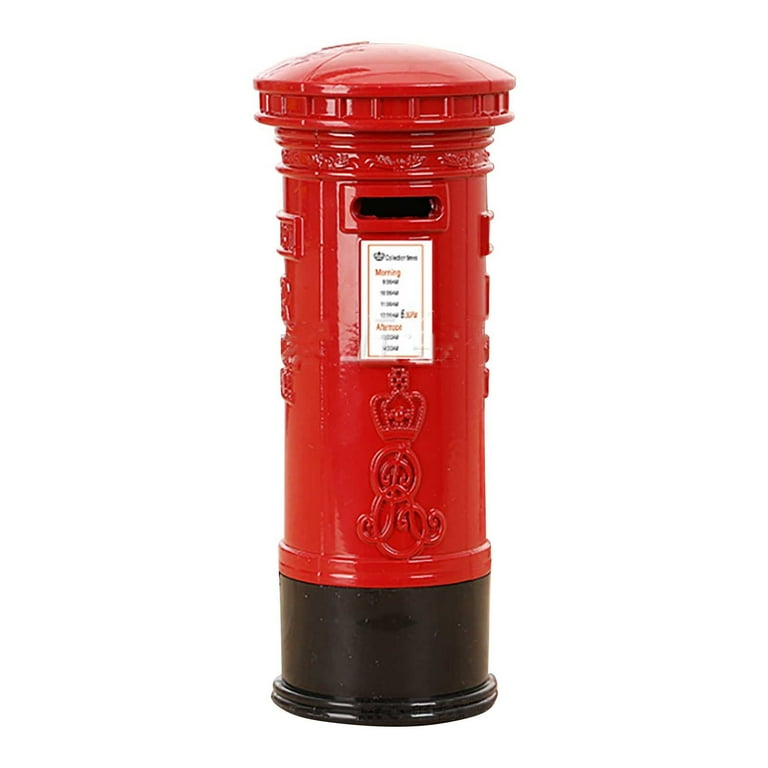The image showcases a cylindrical, vertically-oriented mailbox centrally positioned against a stark white background. This mailbox, characterized by a striking red and black color scheme, features a red upper section capped with a circular, helmet-like top and a black base. Prominently placed on its front is a rectangular white label adorned with small, indistinct blue and red lettering. Below this label, an intricate design is engraved: a crown atop the letter 'R', exhibiting a sophisticated, ornamental style suggestive of British heritage. The functional elements include a horizontal slit near the top for receiving letters. The entire ensemble, marked with its distinct colors and detailed engravings, reflects a traditional postal theme.